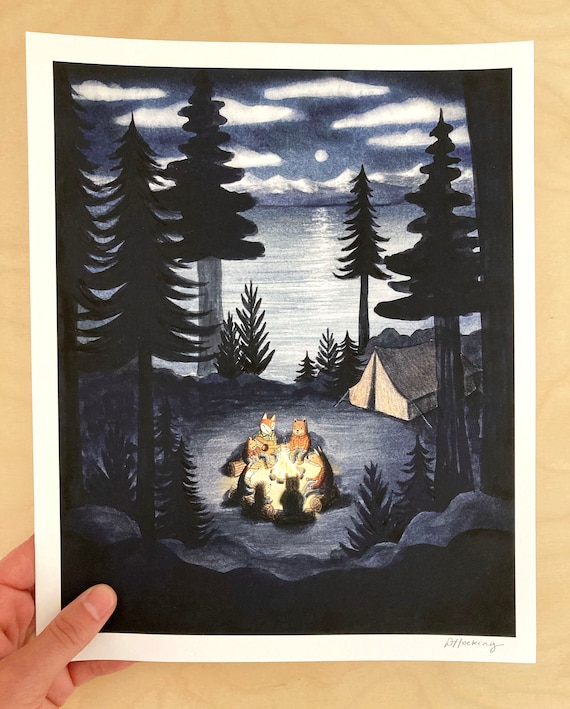In the image, a light-skinned hand holds a large piece of paper against a light wood background, possibly a table. The artwork is a detailed, hand-drawn evening scene featuring a circle of woodland animals gathered around a glowing campfire, with a barely-legible signature at the bottom. The animals depicted include a varied assembly, possibly a fox with a brownish-red head, a reddish-brown bear, potentially a coyote, a kangaroo, and perhaps even Winnie the Pooh. The background showcases a pond or lake that reflects a full moon, which is centered at the top of the drawing among scattered clouds. The moonlight illuminates the scene, casting long, dark silhouettes of rocks and trees in the foreground. Surrounding the animals and their campfire are both small and tall pine trees, enhancing the woodland atmosphere. Just beside the campfire is a sizable beige tent, tinged with darker shades on its sides, adding to the cozy outdoor setting.